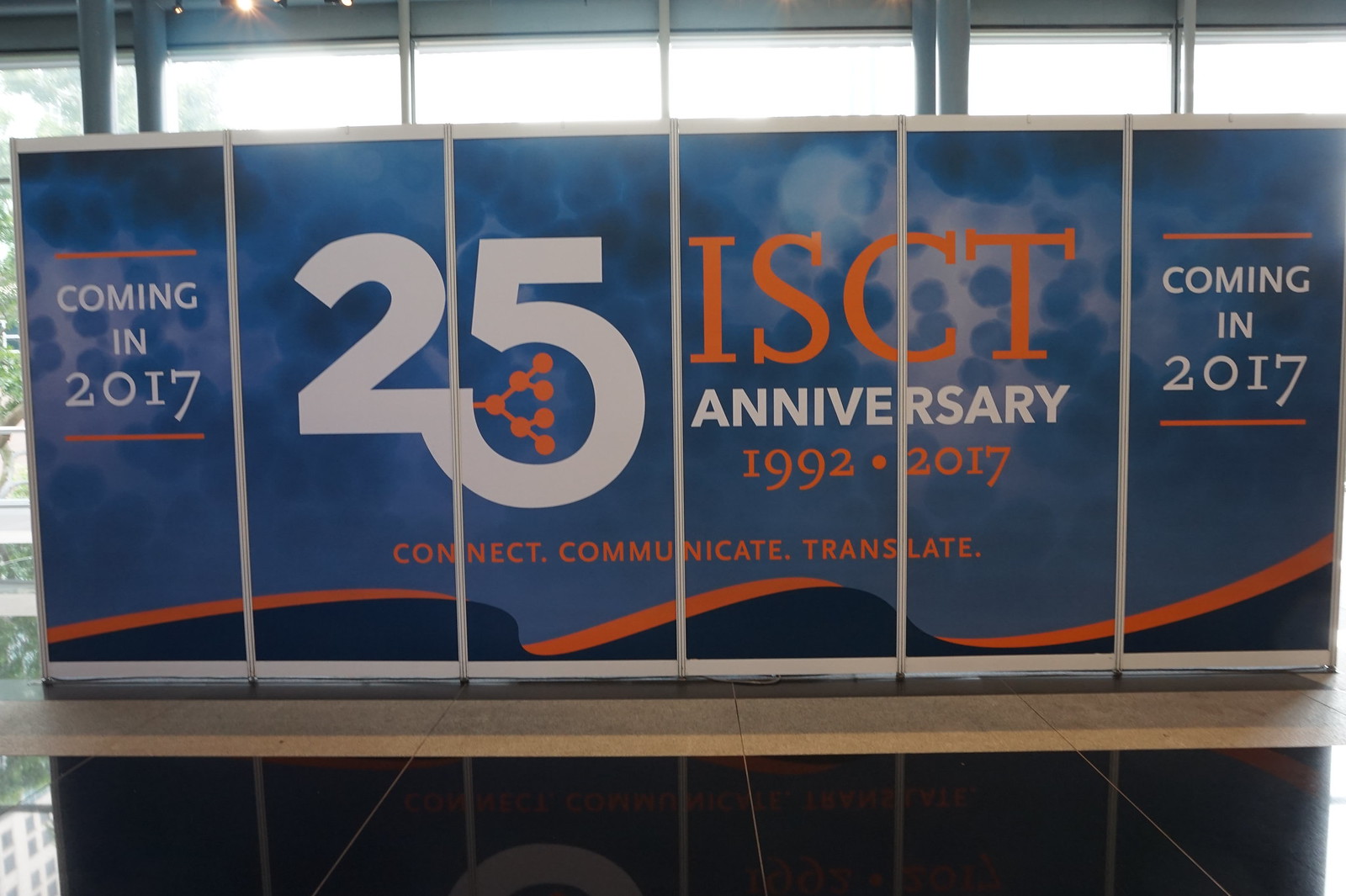In this detailed photograph set inside a large indoor arena with floor-to-ceiling glass windows allowing sunlight to shine through, the main focus is a large sign consisting of six vertically-oriented panels. The floor is a shiny, black glass surface. The panels feature a textured background resembling cloudy, shadowy blue bubbles with a gradient effect. 

The text on the sign prominently displays "25 ISCT Anniversary 1992-2017" across the central four panels, with smaller text below reading "Connect, Communicate, Translate." Both the far left and far right panels repeat the message "Coming in 2017." The letters "ISCT", "1992", "2017", and "Connect, Communicate, Translate" are written in red, while "25" and "Anniversary" are in white. At the bottom of the panels is a decorative element featuring an orange ribbon intertwined with a dark blue one, resembling a genome or hierarchical connection graphic.